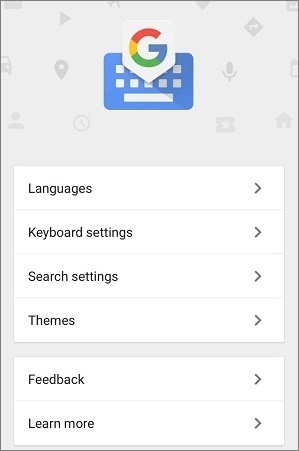This image is a screenshot taken from a Google device, identifiable by the multicolored Google logo centered at the top. The logo, a stylized "G" composed of red, yellow, green, and blue segments, is prominently displayed. Directly below the logo is a blue clip art representation of a keyboard, with contrasting white keys.

Surrounding this central image are various icons associated with Google's services, including symbols for location, microphone, play button, and a clock. Below these icons are clickable options listed in black font on a white background. These options are:

- Languages
- Keyboard settings
- Search settings
- Themes
- Feedback
- Learn more

Each option is accompanied by a right-pointing arrow on its right side, indicating that further action can be taken by selecting these options. The entire layout is minimalist, with a white background and black text, enhancing readability and focus on the content.